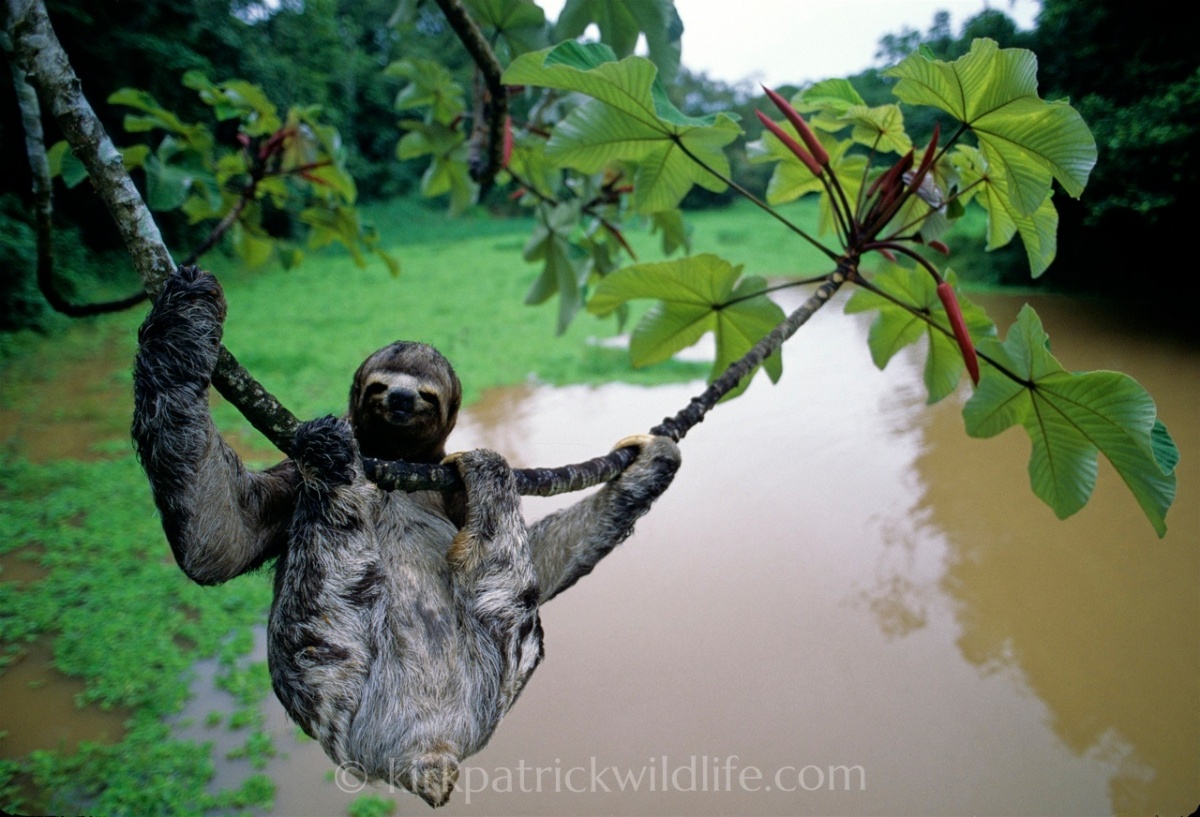This image captures a sloth hanging from a tree branch in a lush, vibrant forest setting. The sloth, with its dark gray fur and tan face, is positioned towards the bottom left of the frame, appearing close—within about five feet. It hangs over a muddy brown river, using both its front claws and back feet to grip the bending branch. The sloth gazes directly at the camera with a gentle smile, almost as if it's posing. Surrounding the sloth, the background is filled with rich greens from the dense foliage. Reds, grays, whites, and hints of black and brown add depth to the scene. At the bottom center of the image, text reads "copyright Kirkpatrickwildlife.com," marking the photo's source.